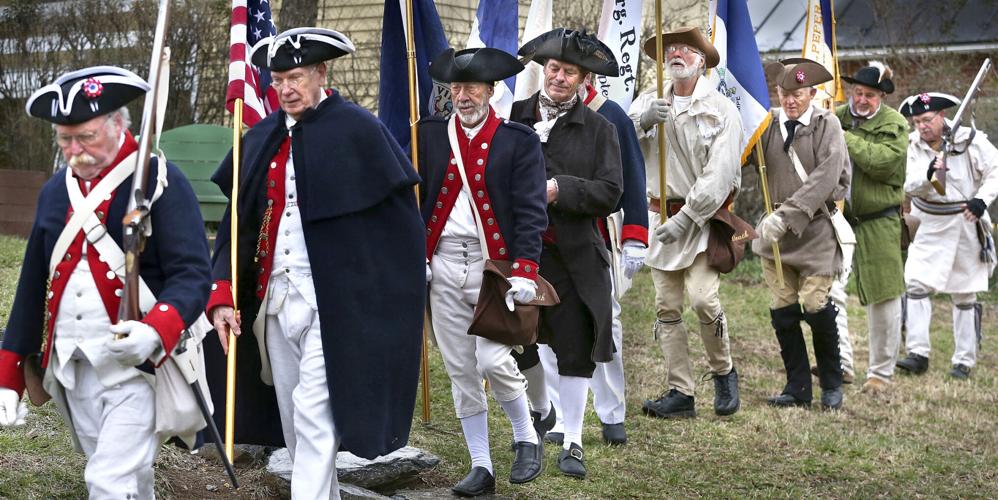This photograph captures an outdoor scene featuring a line of men dressed in American Revolutionary War reenactment uniforms. They stand in a park, their formation extending diagonally across the image from left to right. The men wear distinctive tri-corner hats, blue jackets with red trim, white belts, white pants, and black shoes, with one individual notably in knee-height black boots. The first man holds a rifle in his left hand, while the second carries a flagpole bearing the American flag. Following them, several men also hold flags, except for the last man who holds an old flintlock rifle.

Their uniforms are detailed: blue jackets with red trims, white vests, and white gloves. Some wear blue and white caps, resembling sailor hats. Among the group, one man dons a beige coat and brown pants with brown boots, and another sports a green coat with white pants. In the background, a beige building, leafless trees, a brick wall, and a black-roofed structure are visible. The grass underfoot is a mix of green and dead patches, suggestive of seasonal change. These men are likely participating in a historical reenactment, vividly bringing a bygone era to life.